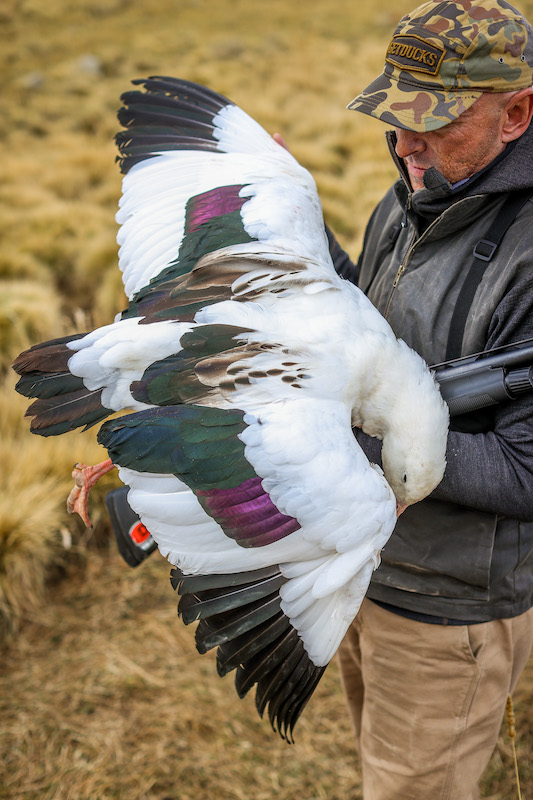This vertical rectangular photograph features a hunter against a blurred background of brown, autumnal grass, indicative of fall. The hunter, appearing to be in his mid-40s with a stubbled face, wears a dark brown leather jacket zipped up against the cold, khaki pants, and a camouflaged cap adorned with the partial, readable inscription about ducks. The cap, in greens, browns, and tan, is slightly turned to the left, obscuring his eyes as he looks down at the sizeable bird he holds.

The bird, recently killed, is primarily white with a three-foot wingspan. Its magnificent feathers display a metallic array of greens, purples, and browns. The wings feature black tips at the edges, and there are brown accents where the wings meet the body. Splashes of metallic green transition into the tail, complemented by purple highlights. The bird's face and neck are white, with an orange bill and webbed feet hinting at a possible duck species. Its head droops lifelessly over the hunter's arm, enhancing the overall somber tone of the image. The photograph, notably taller than it is wide, captures the detailed scene in a visually striking manner.